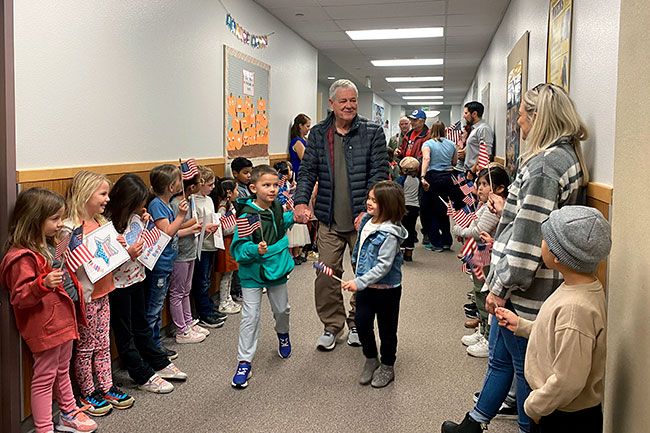The image is a color photograph, rectangular in shape and taken indoors in an elementary school hallway. It captures a vibrant and likely celebratory scene, possibly a Veterans Day event. Children holding small American flags are neatly lined up against the hallway walls, which are paneled halfway down and white at the top portion. Interspersed among the children are parents, adding to the festive atmosphere.

Central to the image is an elderly man with white hair, dressed in a navy blue, down-filled ski jacket over a green buttoned shirt, dark tan pants, and grey running tennis shoes. Flanking him are two young kindergarten-aged children—a girl on his right wearing a grey sweatshirt under a blue denim vest, black pants, and grey shoes, and a boy on his left sporting a green jacket, grey pants, and blue tennis shoes. The man is holding each child by the hand as they walk down the hallway towards the camera.

The hallway is adorned with typical school decor, such as artwork, posters, and framed student art. Other details include a blonde woman in a grey and white striped jacket holding her child’s hand, standing towards the end of the hallway. The overhead fluorescent lights illuminate the scene, contributing to the photographic realism of the image.